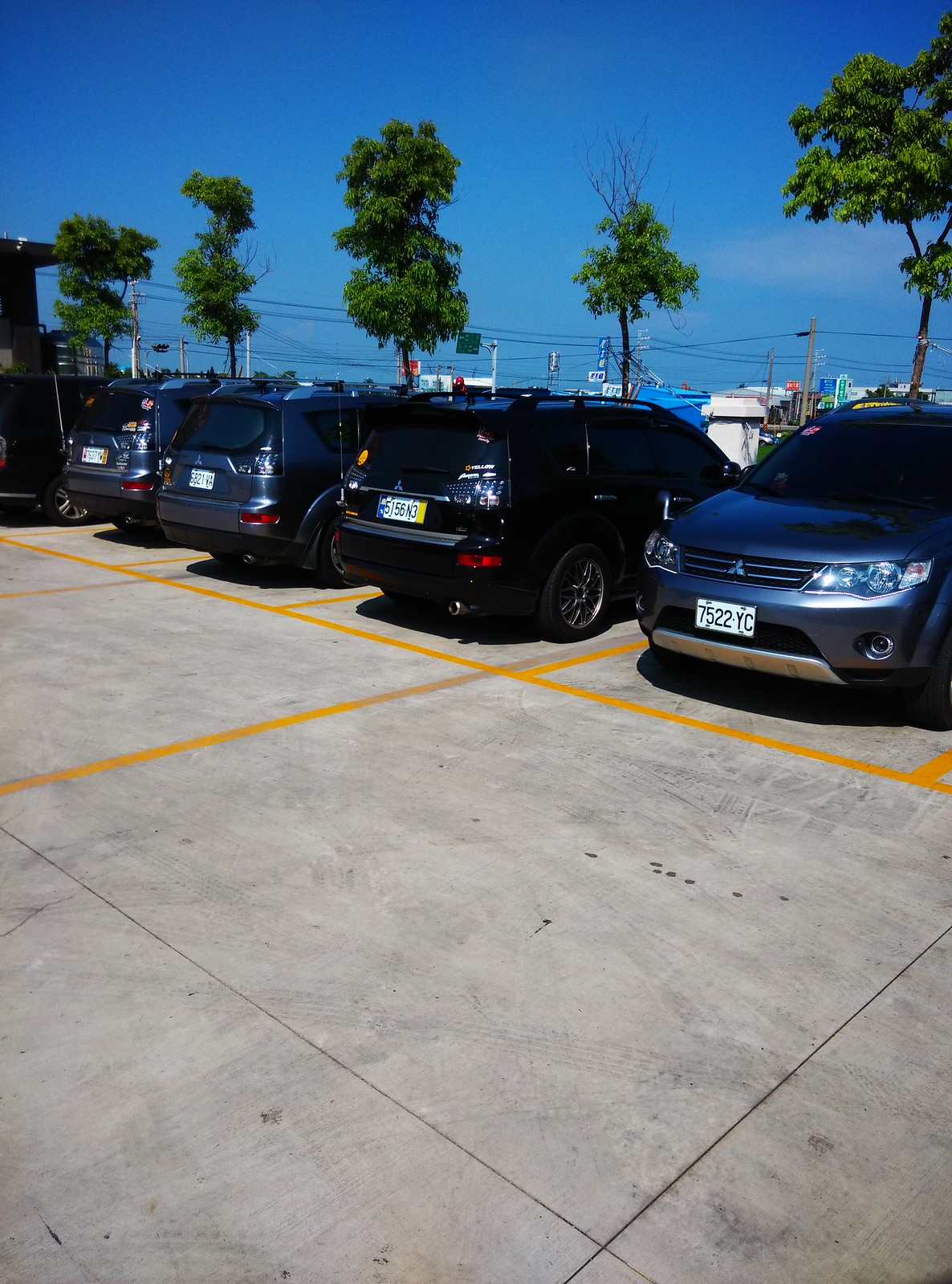This color photo showcases a clear, sunny day in a parking lot, likely near a marina given the presence of what appear to be boats in the background. The blue sky is vibrant, adding to the picturesque quality of the scene. At least five cars, predominantly SUVs and sedans, occupy the parking spaces outlined by yellow lines on the somewhat worn pavement. Among these vehicles, four are parked nose-in, revealing their rear ends, while one Mitsubishi SUV stands out, parked backward with its license plate—7522 YC—clearly visible. All the cars appear to be Mitsubishi models, suggesting the possibility of a dealership or a common event. The background features spindly, young green trees and thin brown trunks, contributing to the airy feel. Power lines in the distance hint at an urban proximity, although the scene retains a tropical ambiance, possibly indicating a location like Florida.